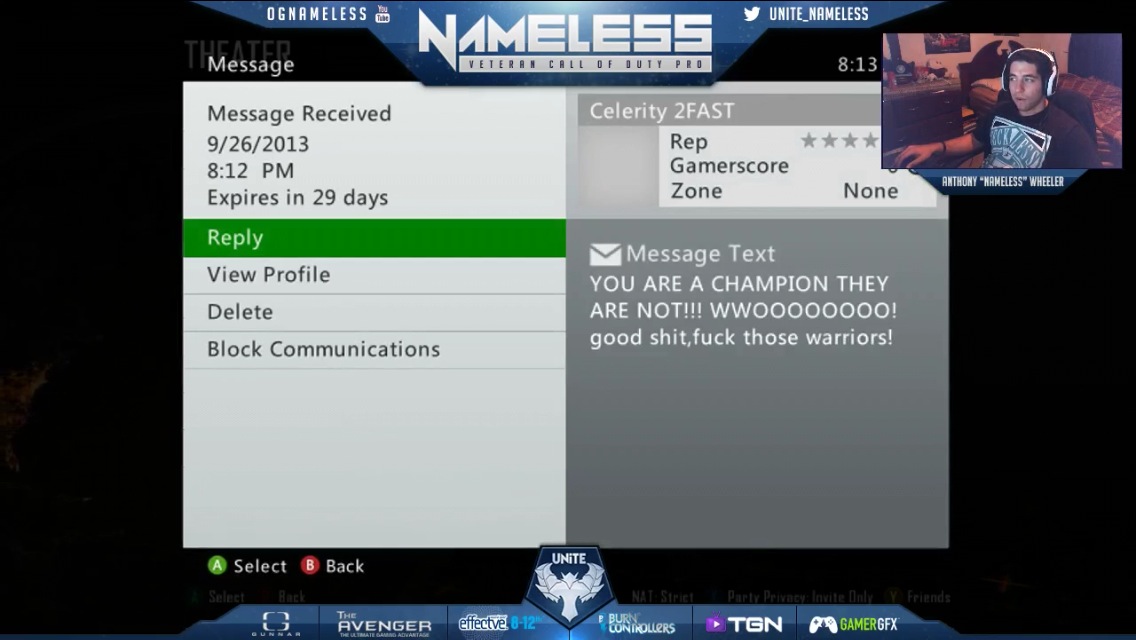Against a dark black background, there's a screen capture from a gamer site featuring a gray message-type board. At the top, a blue banner reads "OG Nameless Nameless Veteran Call of Duty Pro". In the upper right corner is a small image of a player, identified as Anthony "Nameless" Wheeler, sitting behind a desk in his bedroom and wearing white headphones. Below his camera feed, his username is displayed as Anthony "Nameless" Wheeler, along with his Twitter handle, "UNITENAMELESS," and his YouTube channel, "OGNAMELESS."

The message panel under the banner states, "Message received 9-26-2013, 8:12 p.m., expires in 29 days." The message text, reading "You are a champion. They are not. Woo! Good. Shit. F-U-C-K. Those warriors," appears prominently. Below the text, options such as "Reply," "View Profile," "Delete," and "Block Communications" are indicated, with "Reply" highlighted in green. Additional green writing and several logos can be seen at the bottom of the screen.